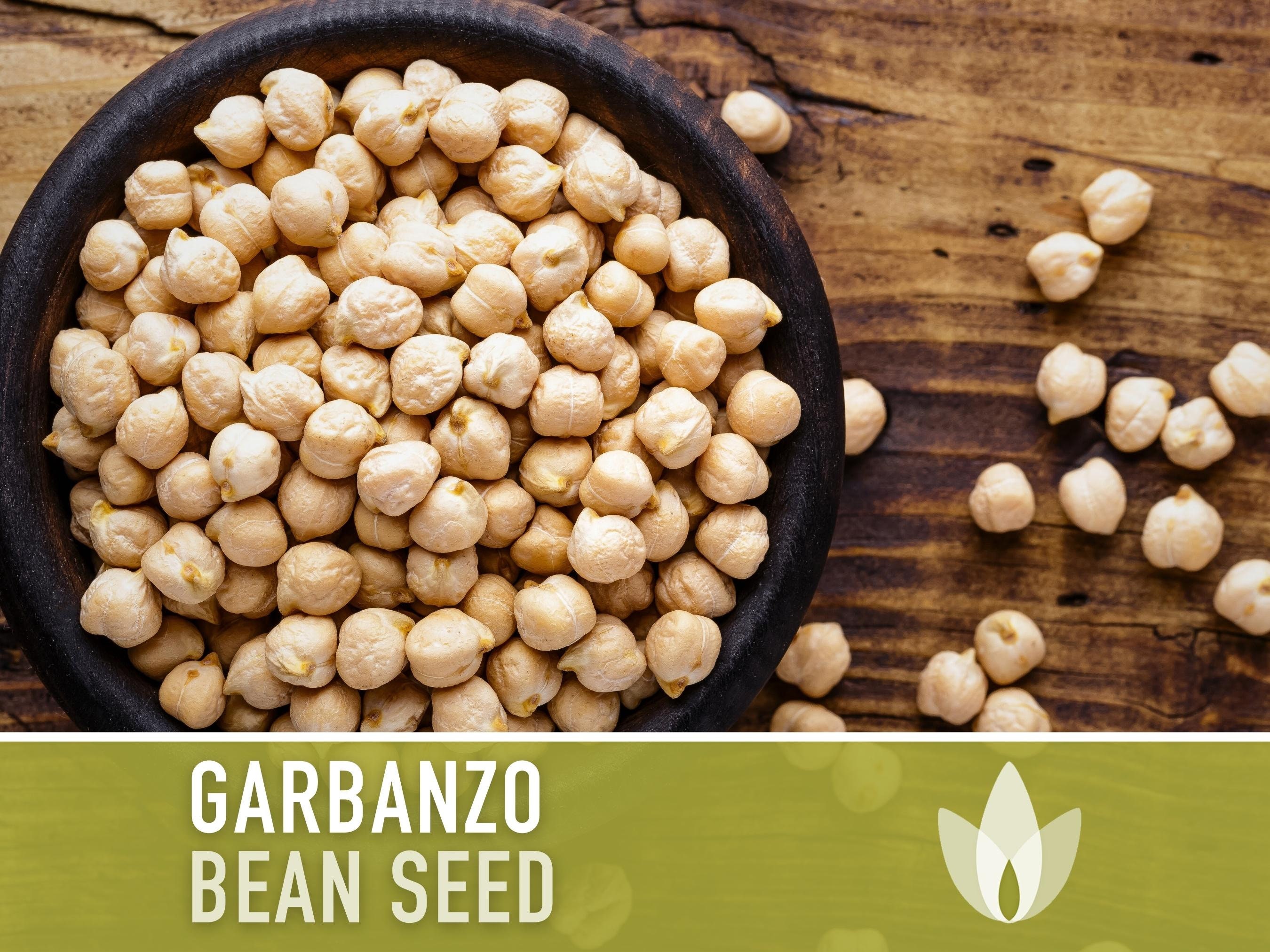This top-down photo captures a rustic wooden table featuring a dark, wooden bowl filled to the brim with garbanzo bean seeds. The seeds, resembling small, pale brown to whitish nuts, have a textured, bumpy surface and vary subtly in shade due to the light source. Some seeds have spilled onto the table, adding a touch of organic imperfection. At the bottom of the image, a greenish, transparent banner displays the words "Garbanzo Bean Seed" in white text, accompanied by an illustration of overlapping leaves. The table itself, with its rich brown, tan, and dark brown grain, provides a natural and earthy setting, complementing the deep, dark wooden bowl and its contents.